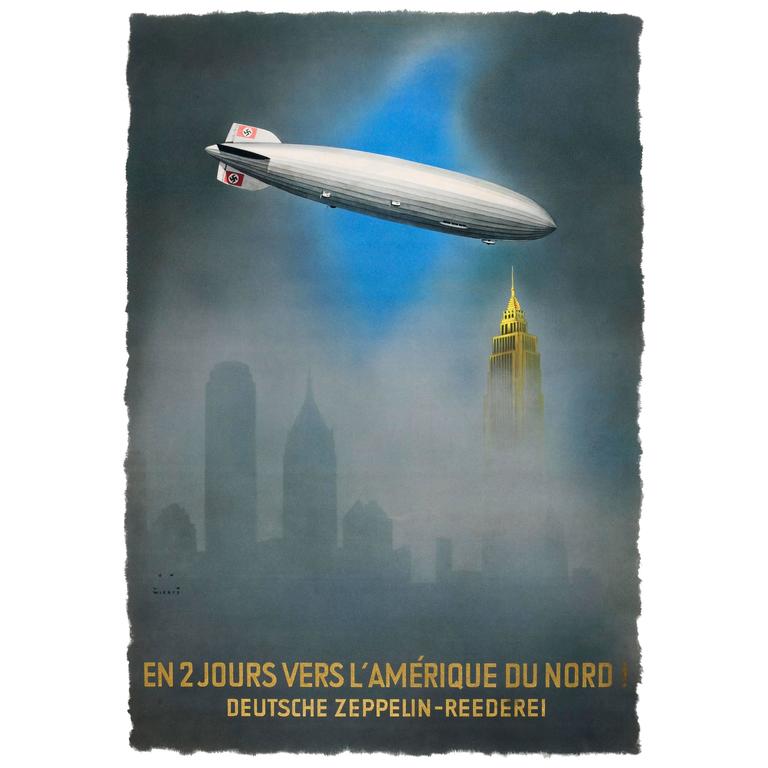This is a vertical rectangular poster with rough, irregular edges. Dominating the scene is a silver Zeppelin flying through a hazy, foggy sky. Its position seems somewhat descending, and it prominently features German swastikas on its tail. Behind the Zeppelin, a patch of dark blue sky contrasts with the otherwise opaque atmosphere. Below the Zeppelin’s nose, the top of a grand building with a gold dome is visible, reminiscent of, but not necessarily, the Empire State Building. The cityscape is filled with vague outlines of other tall, gray buildings emerging through the haze, giving the impression of a large metropolis. At the bottom of the image, there is text written in French in gold letters, adding an elegant touch to the overall composition.